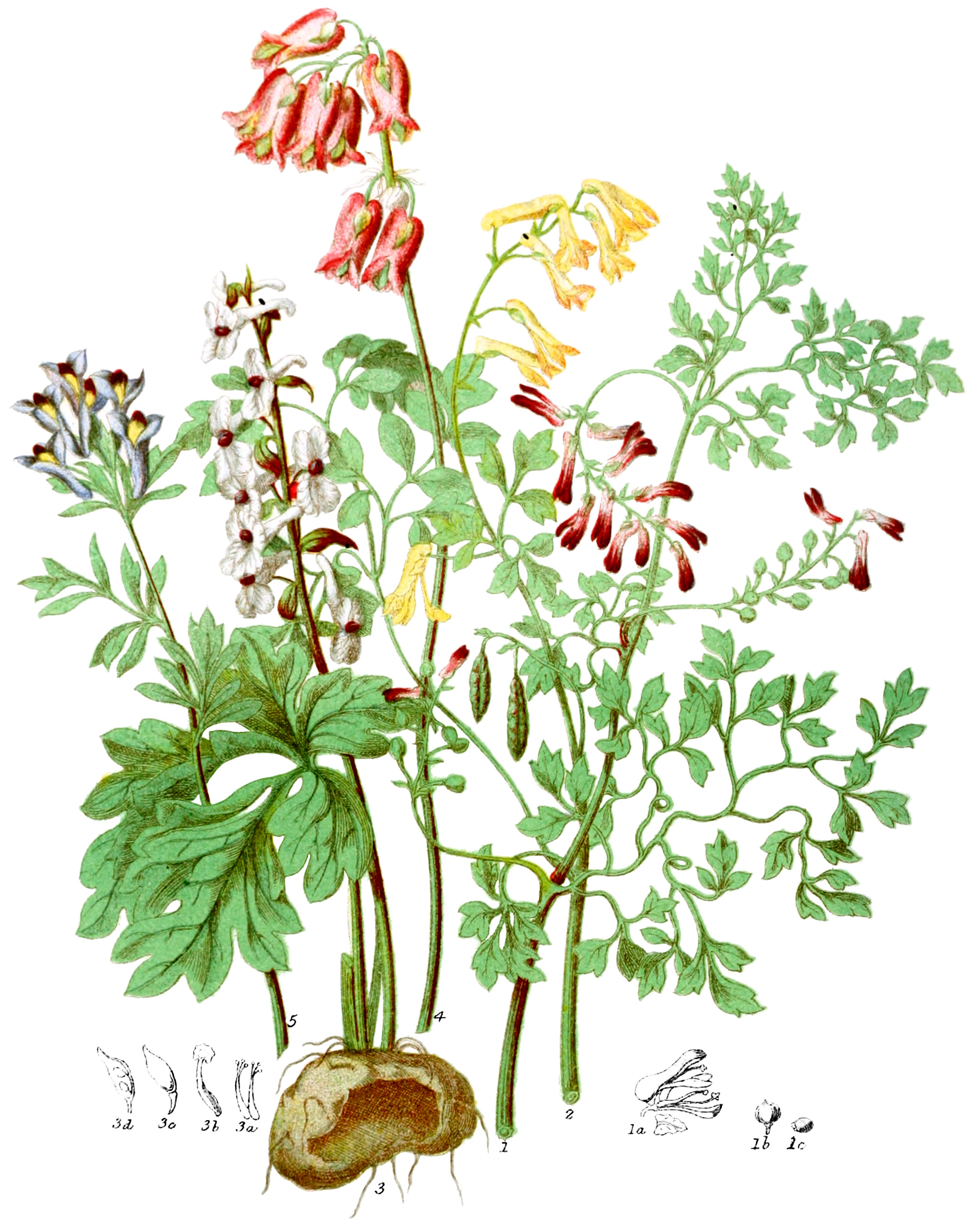This detailed illustration depicts a variety of long-stemmed flowers and botanical elements against a white background. Prominently featured are tall, vibrant flowers including pink, yellow, and a deep shade of purple that haven’t quite opened. Complementing these are delicate white and blue bell-shaped flowers, perhaps bluebells, gracefully hanging in the air. Dense green foliage anchors the composition, wrapping around the various blossoms. 

At the bottom of the image, a brown sack-like object, with an opening possibly resembling a hacky sack, adds an earthy element to the scene. Surrounding this brown object are several smaller, detailed black and white botanical sketches. On the bottom left, labeled 3D, 3O, 3B, and 3A, are intricate images, including a small bulb, a piece that appears to be a mushroom, and two baby carrots with sprouting hair. On the bottom right, labeled 1A, 1B, and 1C, the images include a variety of mushrooms, a pollen bulb, and a small nut.

Numerical markers (5, 3, 4, 1, 2) guide the viewer from left to right across the center of the illustration, highlighting a progression of flowers: a prominent purple flower, white blossoms on a long stem, dripping red bell flowers, followed by yellow bell flowers, leading to varieties of red and white flowers. The scene emphasizes the stages of blossoming, with some flowers in a budding phase and others more fully opened, underscoring the rich diversity of plant life illustrated in this detailed and educational sketch.